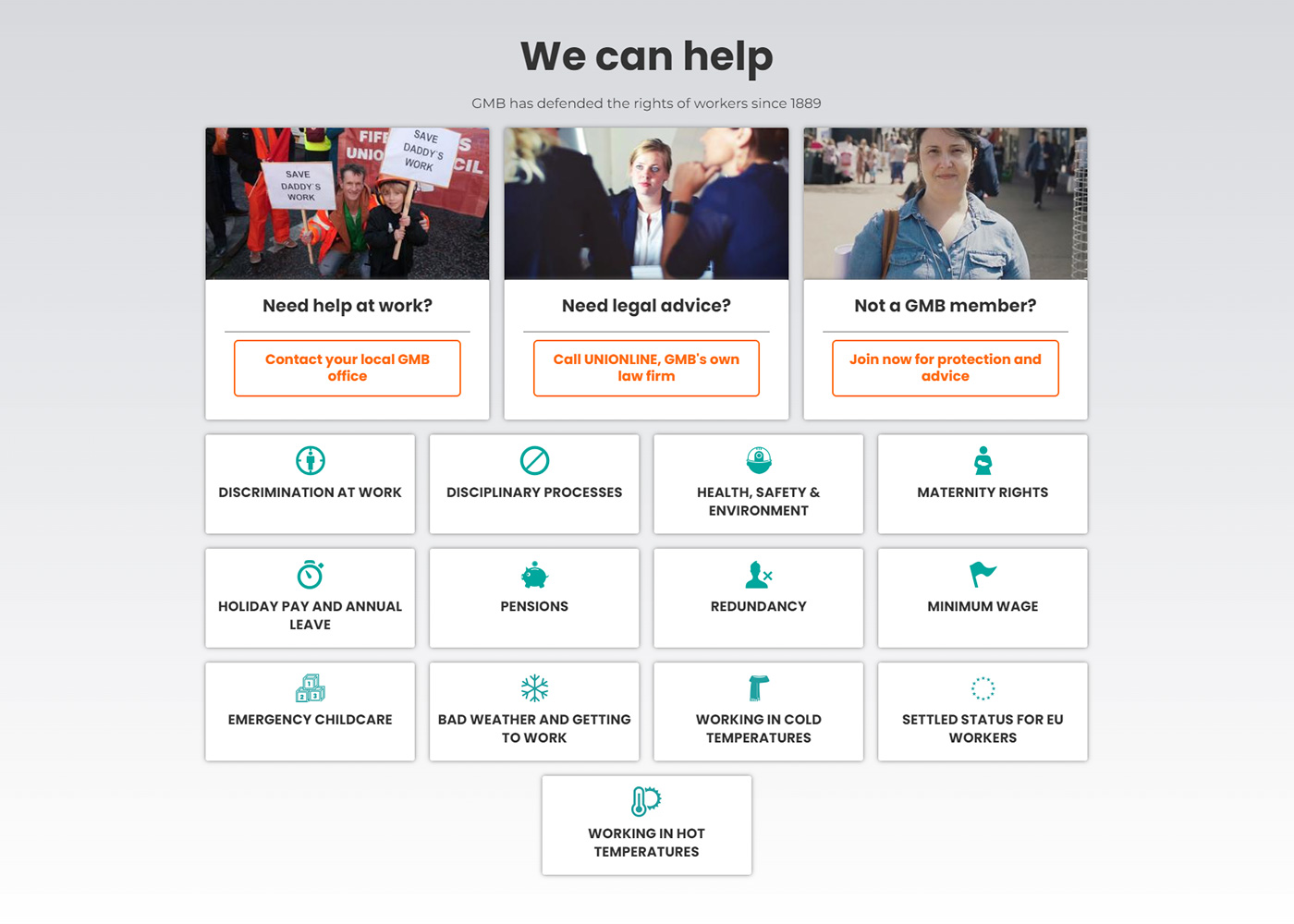**Caption:**

On a gradient gray background that transitions from darker gray at the top to white at the bottom, a prominent black message reads "We can help" in the middle-top section. Beneath it, in a slightly darker gray text, is the statement "CMB has defended the rights of workers since 1889."

Below this message, three images are presented, each with an orange-outlined button beneath them. The first image depicts people holding signs, paired with a button labeled "Need help at work" leading to "Contact your local GMB office." The second image shows two individuals conversing and a third looking nervous, paired with the button "Need legal advice" that directs to "GMB's own law firm." The third image features a woman in a jean jacket with the text "Not a GMB member?" and a button prompting "Join now for protection and advice."

Following this, a three-by-four grid of buttons is displayed, each featuring green icons on white backgrounds accompanied by black text. These buttons provide quick access to essential worker information such as "Emergency childcare," "Redundancy," "Pensions," "Holiday pay," "Maternity rights," "Retired settled status for EU workers," "Working in hot temperatures," and "Disciplinary processes."

This layout is part of a website for a union that offers its members a portal to easily obtain crucial information and resources regarding their employment rights and benefits.